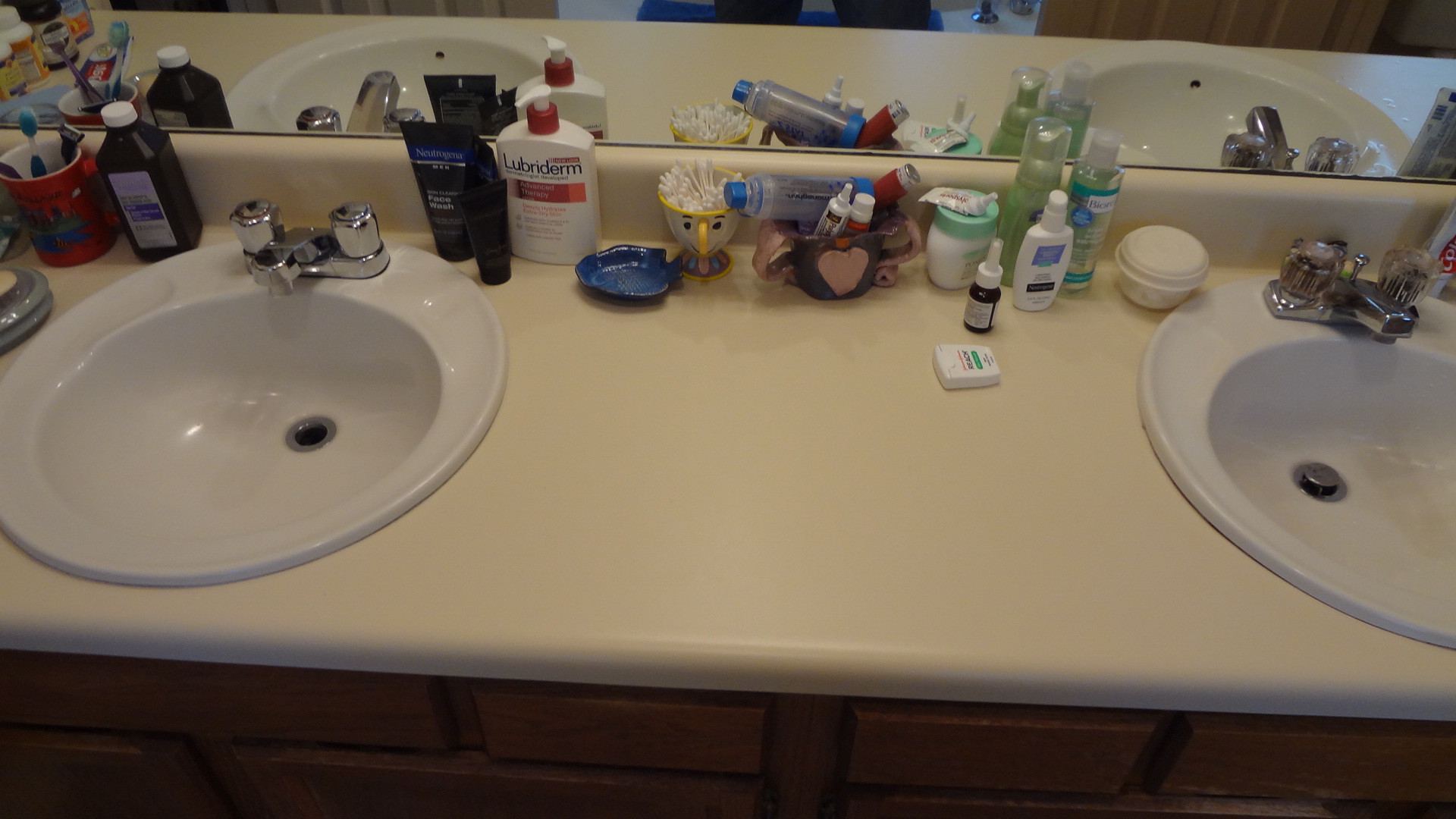This photograph captures a section of a household bathroom featuring a spacious beige countertop with wooden cabinets and drawers beneath. The countertop houses two round white sinks, each equipped with identical faucets that include dual knobs and a short spout. Notably, the sinks are positioned several feet apart but share the same countertop for a clean and cohesive design. 

Above the sinks, a large mirror extends across the wall, reflecting the bathroom's details. The countertop itself is cluttered with a variety of personal care items. From left to right, you can see a cup containing toothbrushes, a black bottle of peroxide, several tubes of products, a lotion bottle, a cup filled with Q-tips, and a container of floss. The assortment of products suggests a busy, well-used space, characteristic of daily personal grooming routines.